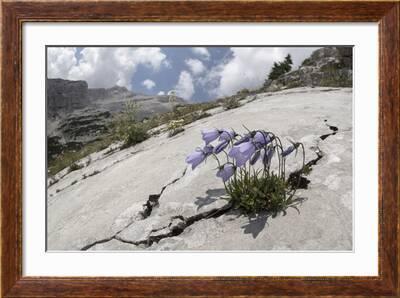A detailed photograph within a dark wooden frame captures a serene yet striking natural scene. The inner background of the frame is matte white, providing a stark contrast to the vivid photograph it holds. The focal point of the image is a rugged, light gray mountainside with a prominent crack. Emerging from this crack are delicate light purple flowers, their trumpet-like blooms resembling tulips, supported by green stalks and grass-like greenery. The photograph is set in a landscape orientation, with the greys and greens of the mountains extending into the distance. In the background, additional mountain ranges can be seen, dotted with sparse trees and bushes. Above, a light blue sky, heavily covered with clouds, suggests a slightly cloudy morning. This vibrant yet peaceful scene beautifully captures the resilience of nature amidst the harshness of the rocky terrain.